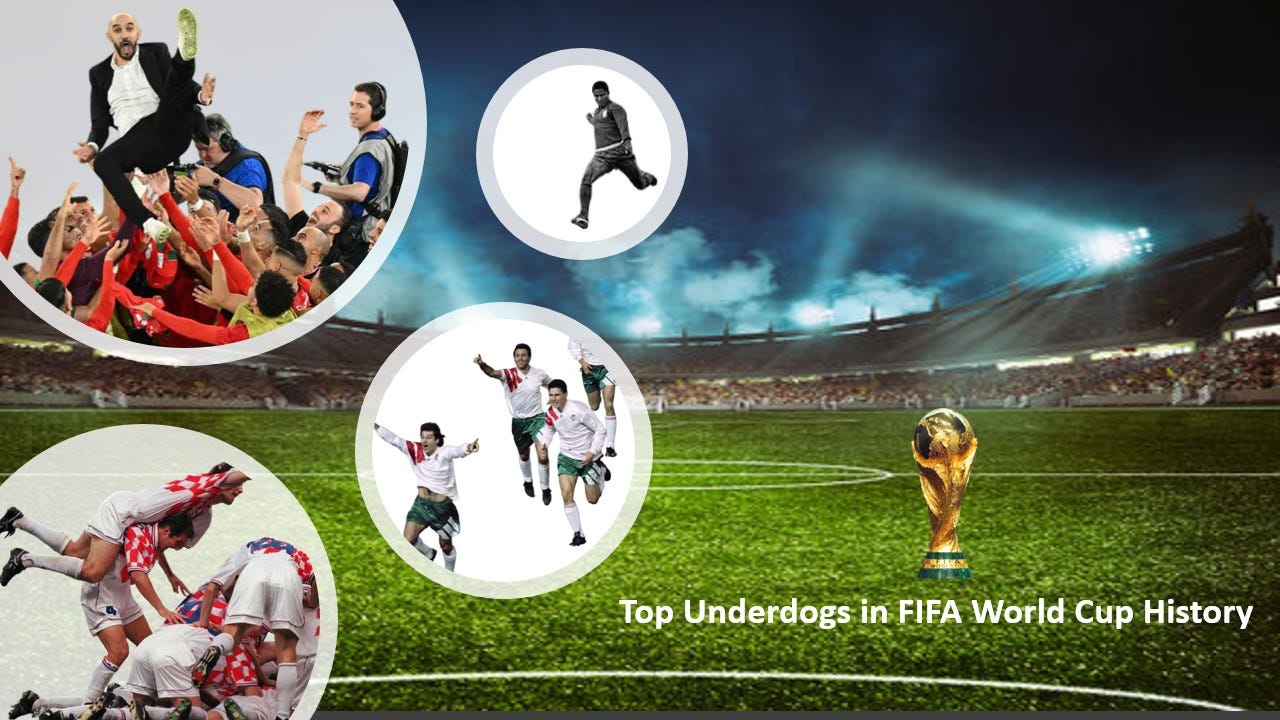The image captures a vivid nighttime scene at a soccer stadium filled to capacity with enthusiastic spectators. The sky is cloaked in deep blue hues, punctuated by ominous grayish-blue clouds, and illuminated by bright stadium lights that cast spotlight beams onto the vibrant green soccer field below. The stadium, a grand structure, looms in the background, alive with energy.

In the bottom right corner, white text reading "Top Underdogs in FIFA World Cup History" is prominently displayed next to a gleaming golden trophy, presumably awarded to the World Cup champions.

On the left side of the image, there are four white circles with gray outlines, each containing photos of celebratory moments. The top left circle is the largest and features a coach in a black suit, white shirt, and green shoes being lifted by his jubilant team clad in red. The top right circle shows a black and white image of a player mid-run, left leg forward. The bottom left circle displays a team of players in white jerseys with red stripes and green shorts celebrating, while the bottom right circle depicts players in red and white shirts and white shorts piling on each other in victory.

These visuals collectively narrate the triumphant story of a team that emerged as one of the greatest underdogs in FIFA World Cup history, immortalizing their indomitable spirit and memorable victory.